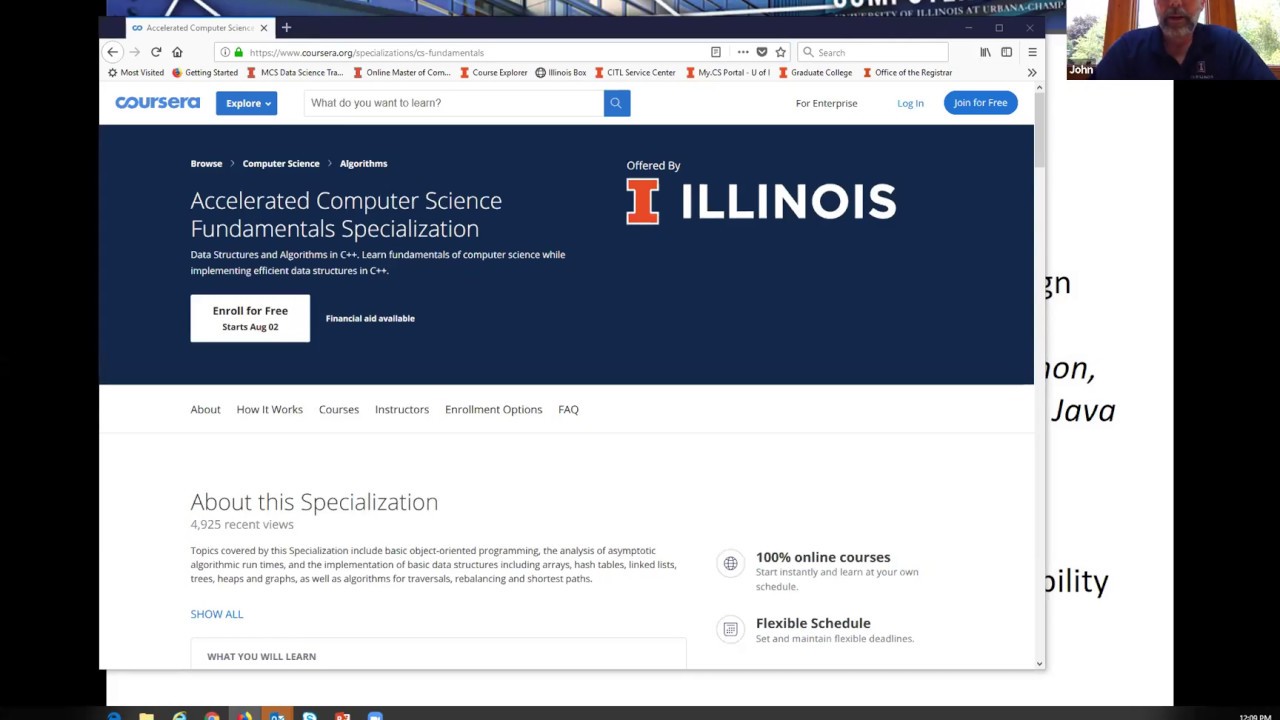On the web page, Coursera presents the "Accelerated Computer Science Fundamentals Specialization," developed by the University of Illinois. The university's logo features a capital red "I" beside the word "Illinois" in white lettering. The page highlights that you can "Enroll for Free," with courses starting on August 2nd, and emphasizes that the program is an online course with a flexible schedule. There is a small section with tiny text summarizing details about the specialization and an option to "Show All" for additional information. The bottom half of the webpage has a white background and appears to be overlaid on what might have been an email, as the word "Java" is visible beneath the overlay. The webpage also includes several headings, such as "How it Works," "Courses," "Instructors," "Enrollment Options," and "FAQ," for easy navigation.